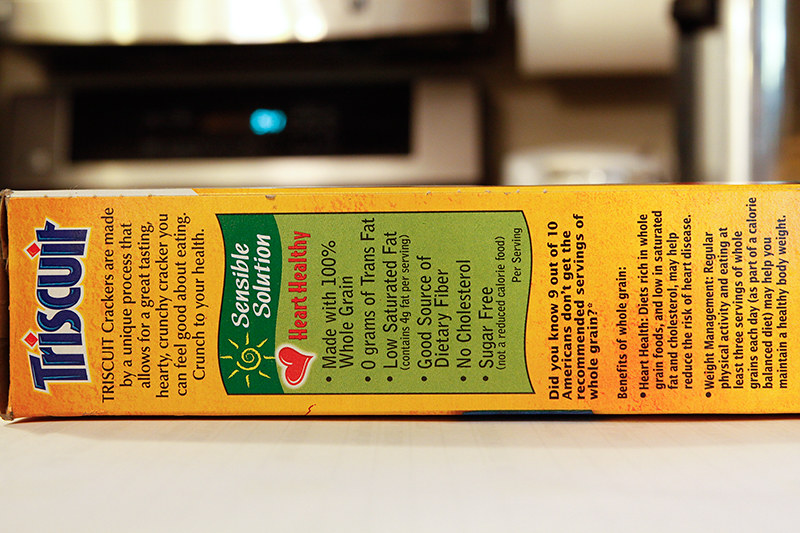The image depicts a box of Triscuits laying on its side on a white surface. The box is positioned with the top facing towards the left side of the image. The trademark "Triscuit" is prominently displayed in blue letters on the top of the box, while the box itself is primarily yellow with a substantial amount of black text. A green label is visible on the box, along with a "Heart Healthy" sign represented by a red heart, featuring the words "Heart Healthy" in red letters nearby. Additionally, the phrases "Sensible Snacking Solution" are written in white letters. The side of the box includes various details, possibly ingredients and other information. In the blurred background, a kitchen setting is discernible with what appears to be a metal coffee pot and either a microwave oven or a toaster oven.